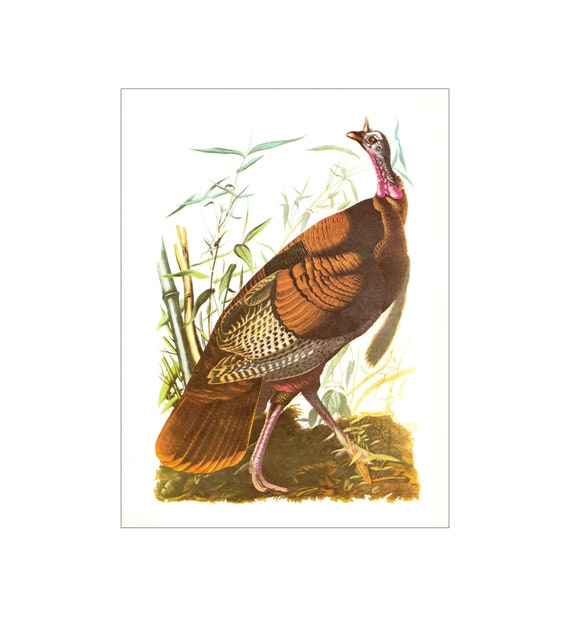The image is an old-fashioned, colorful illustration of a wild turkey in motion, appearing to walk through a mix of brown earth and green foliage. The turkey is predominantly brown with a small white head and a red throat. Its body features a mix of brown, black, and white feathers, particularly on its wings and abdomen where there are spotted patterns. The bird's neck is not very long but it is skinny, leading to a brown beak. It is positioned with its head turned sideways, looking back as if squawking, and its legs, which are purplish-brown and slim, are outstretched, giving a sense of motion. Surrounding the turkey, there are bamboo-like plants and various green leaves, adding depth and a natural setting to the background.